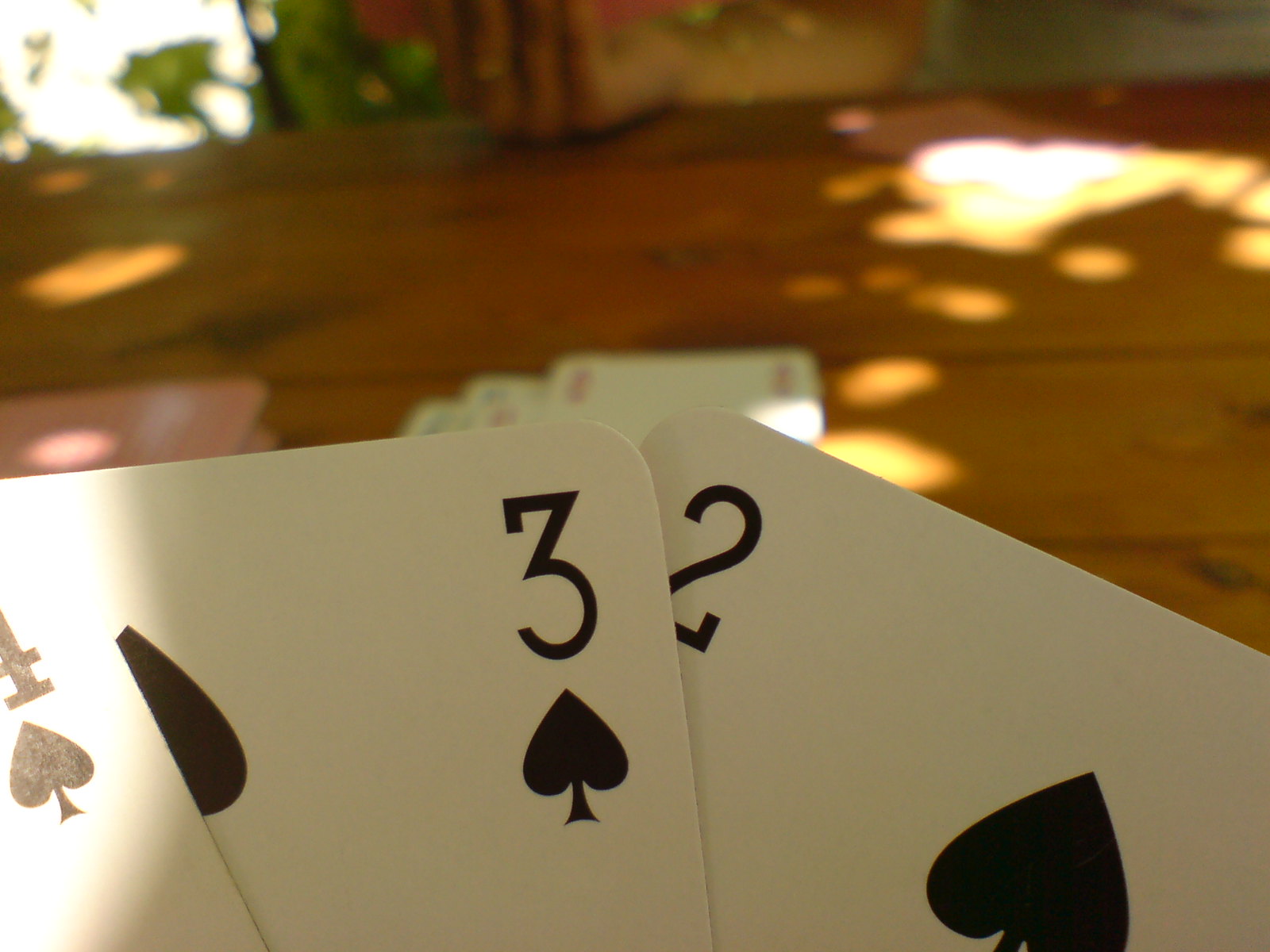The image features a close-up view of three playing cards laid out on a stained pine wood table, bathed in natural sunlight. The table, stained a light golden brown with slightly darker tones at the back, features random, circular splotches of sunlight. In the background, on the left side, a portion of a window can be seen, with bright light shining through and illuminating the edges of green leaves.

In the forefront, prominently displayed, is the three of spades in black lettering, positioned centrally between two other cards. To the right is the two of spades, while to the left, only partially visible, is the four of spades. The sunlight causes the black spade symbols to appear almost gray.

Further back on the table, the blurred image reveals at least three more cards—possibly four—scattered and slightly overlapping. Among them, three cards exhibit red hues, indicative of hearts or diamonds, while another black card is discernible to the left.